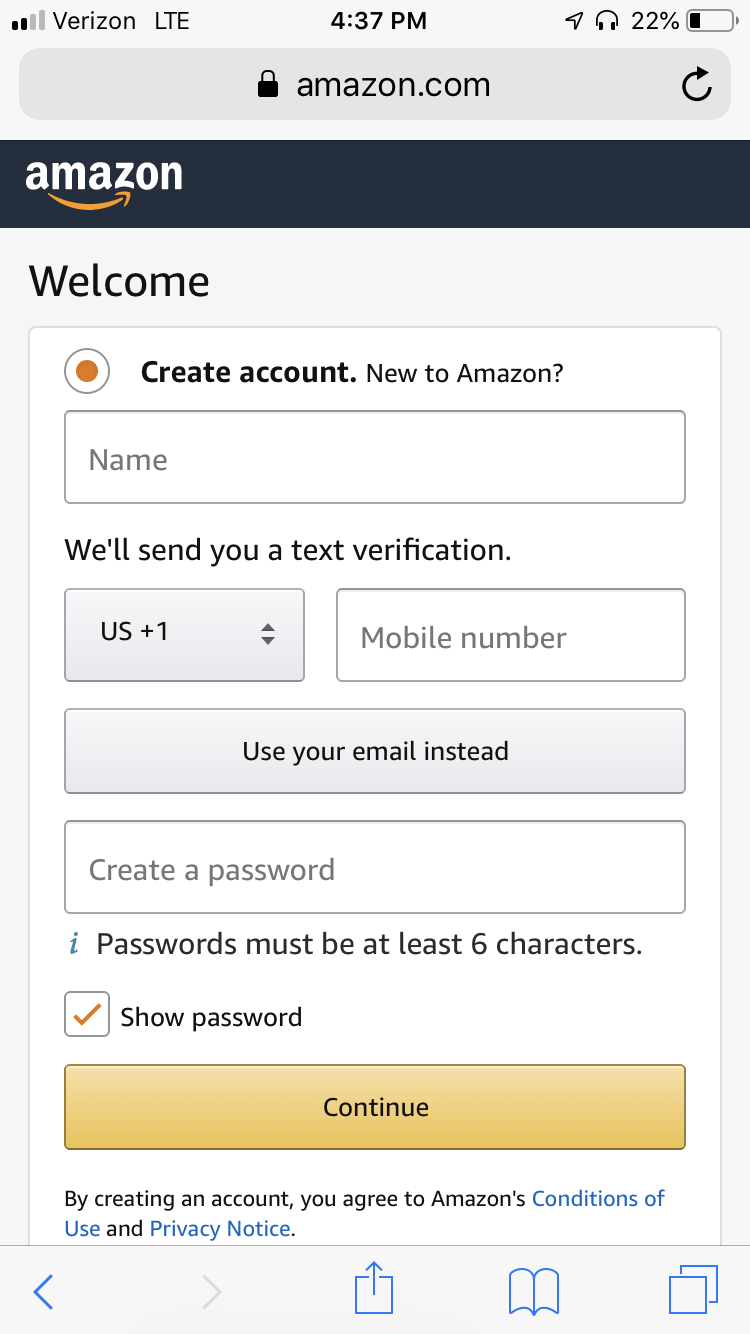*On an iPhone with Safari browser, someone is on the Amazon mobile site creating a new account. The screen displays the "Welcome, create account" page, which prompts the user to enter their name, phone number or email for verification, and create a password that must be at least six characters long. A checkbox is available to choose whether or not to show the password as it is being typed. Currently, no information has been entered. A prominent yellow "Continue" button is displayed at the bottom. The page also notes that by creating an account, the user agrees to Amazon's conditions of use and privacy notice. The interface feels distinctly Amazon-like, featuring a dark blue or black band at the top with the Amazon logo visible. The phone's status bar shows a 22% battery level, headphones plugged in, and an LTE connection instead of Wi-Fi. The default country code for the phone number is set to +1, indicating a US-based phone number, but this can be changed if needed.*